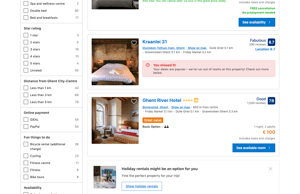This image appears to be a screenshot from a hotel booking website. The quality is poor, making the text difficult to read and more blurry upon zooming in. On the left-hand side, there is a set of filtering options that users can select to narrow their search. The first visible option allows users to filter hotel choices by star rating, with categories for one-star through five-star ratings. Below that is another filtering option with indistinct label text, followed by two more choices, the last of which pertains to activities or amenities ("things to do"), offering specific clickable options to refine the search further.

On the right-hand side of the screenshot, results for two hotel searches are displayed. The first result shows an image of a hotel room with a bed featuring white sheets and a dark headboard. The name of this hotel appears to be "Hotel 31," although the text is very unclear. The second result shows a room with two large windows and what appears to be a bed. This hotel seems to have a name that includes the word "River," but again, the text is largely unreadable.